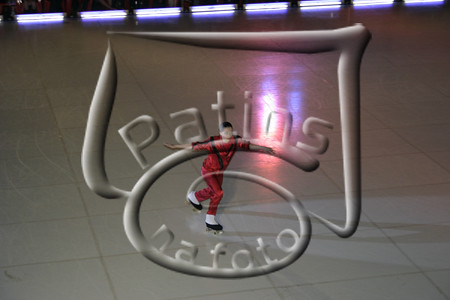The image depicts a digitally rendered scene of a male roller skater, situated in the center of an empty roller rink with a smooth white tile floor, delineated by tan lines that divide it into regular rectangles. The skater is dressed in a matching red outfit comprising a short-sleeve top and long pants, adorned with a distinctive black V-shaped diagonal stripe. He is sporting black and white roller skates, identifiable by the wheels and the front brake on the toe, confirming they are roller skates rather than ice skates or roller blades. The floor around him is expansive and empty, and the scene is illuminated by overhead lighting, creating a glare on the floor. Overhead, there is a border or fencing-like structure. A watermark on the image reads "Patios Nefoto," suggesting ownership or photography credit. The resemblance of the skater's outfit to Michael Jackson's "Thriller" attire adds a touch of nostalgic flair to the visual.